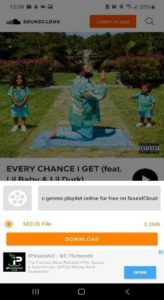In this grainy and blurred screenshot of a mobile device, the SoundCloud app is visible in the background. The time displayed on the device reads 12:39, and the battery percentage appears to be between 50% and 55%. At the top right corner of the screen, there is a magnifying glass icon signifying the search bar. The SoundCloud logo is prominently visible. The screen appears to show a track that includes three individuals: a man and two children, and possibly features the song "Every Chance I Get" by Lil Baby and Lil Durk. Additionally, there is a reference to a music file size of 2.2 MB available for download. At the bottom of the screen, the usual navigation buttons are present: recent apps, home key, and the back button, arranged in their standard order.